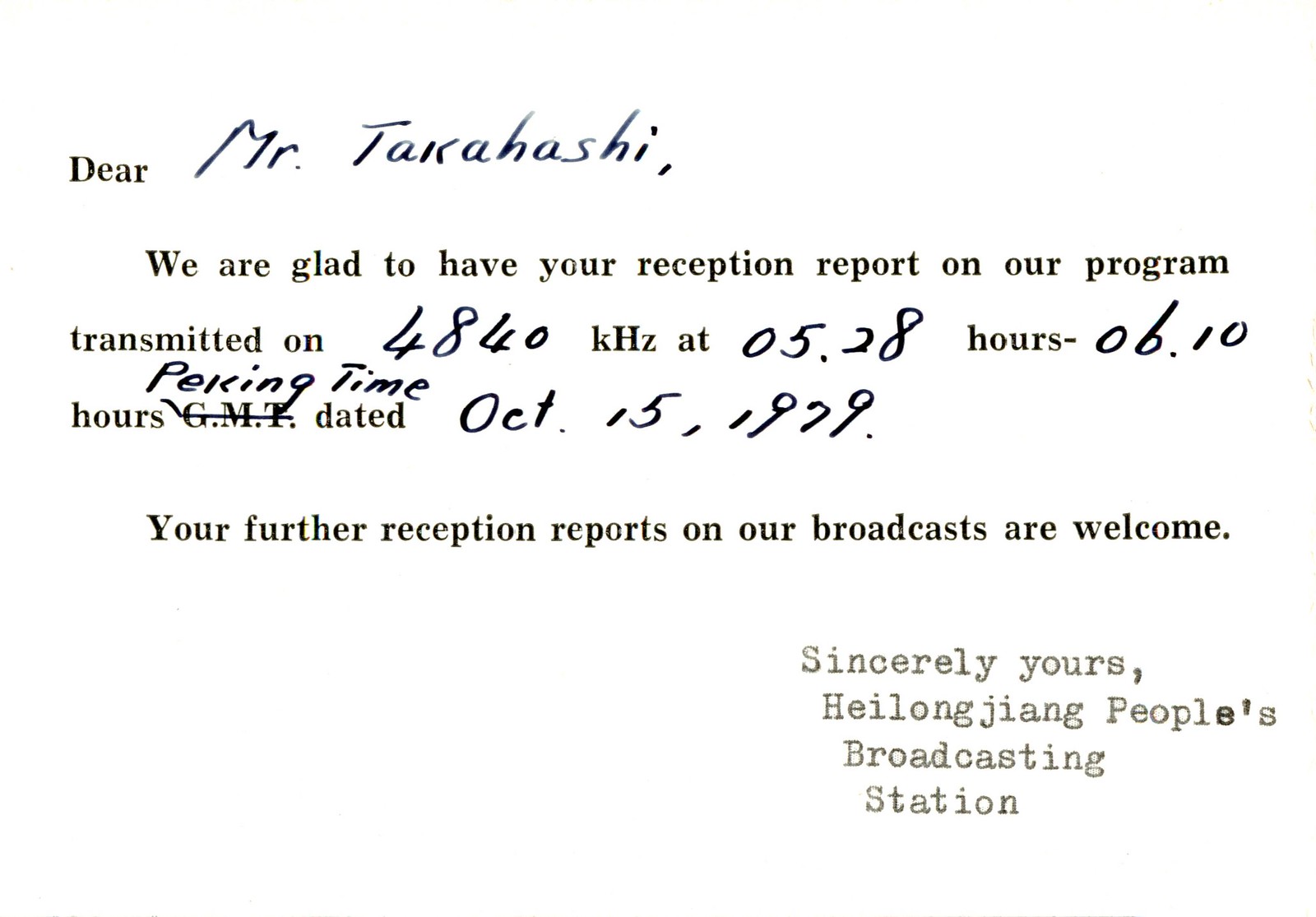The image is a photograph of a form letter addressed to Mr. Takahashi. The letter begins with "Dear," typed in black text on a white background, followed by "Mr. Takahashi" handwritten in black ink. The first paragraph reads: "We are glad to have your reception report on our program transmitted on 4840 kHz at 05.28 hours - 06.10 hours Peking time." Notably, "Peking time" is handwritten and overwrites the originally typed "GMT." The date, "October 15, 1979," is handwritten in black ink as well. The second paragraph continues in typed text: "Your further reception reports on our broadcasts are welcome." The closing section, located towards the lower right of the image, is typed: "Sincerely Yours," followed by "Heilongjiang People's Broadcasting Station," with the station's name typed in a different font and a lighter gray ink. All handwritten elements fill in predetermined gaps left by the typed template.